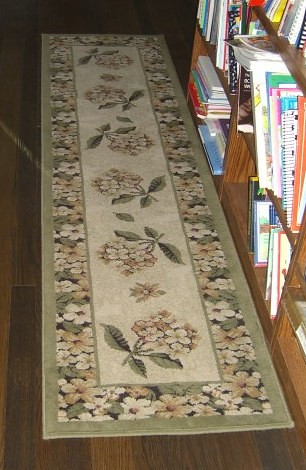The photograph captures a room featuring a wooden floor with a long, narrow runner rug prominently displayed. The rug is characterized by a detailed series of borders and patterns: a light olive-green outer border, followed by a thicker border adorned with a floral design in shades of green, whites, browns, and a dark mustard yellow. The central panel of the rug is beige, decorated with pinkish-brown and white flowers with green leaves. Adjacent to the rug on the right is a medium to dark brown wooden bookshelf. The bookshelf has at least three shelves, filled with a variety of books in different colors such as white, green, pink, red, and blue, arranged both vertically and horizontally, with some books leaning at various angles.